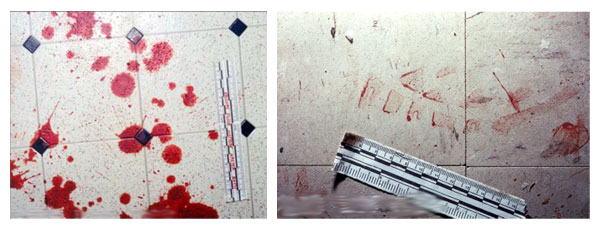The image comprises two small square photos separated by a white line, both depicting details from a probable crime scene with evident blood spatter. The left image shows an overhead view of a white tile floor, characterized by a pattern of black diamonds at the intersections of the tiles. Blood spatter is noticeable across the floor, with various splotches and droplets prominently displayed. A small vertical ruler is positioned on the left side, aiding in the scale measurement. The right image features a cream-colored ceramic tile floor with smeared and scattered blood, indicating possible partial cleaning. At the bottom of this image lies a silver ruler with black markings. Amidst the tiles, there are additional black specks and faint fingerprints visible in the blood smears. Both images present a detailed forensic overview of the blood patterns and the scene's details.